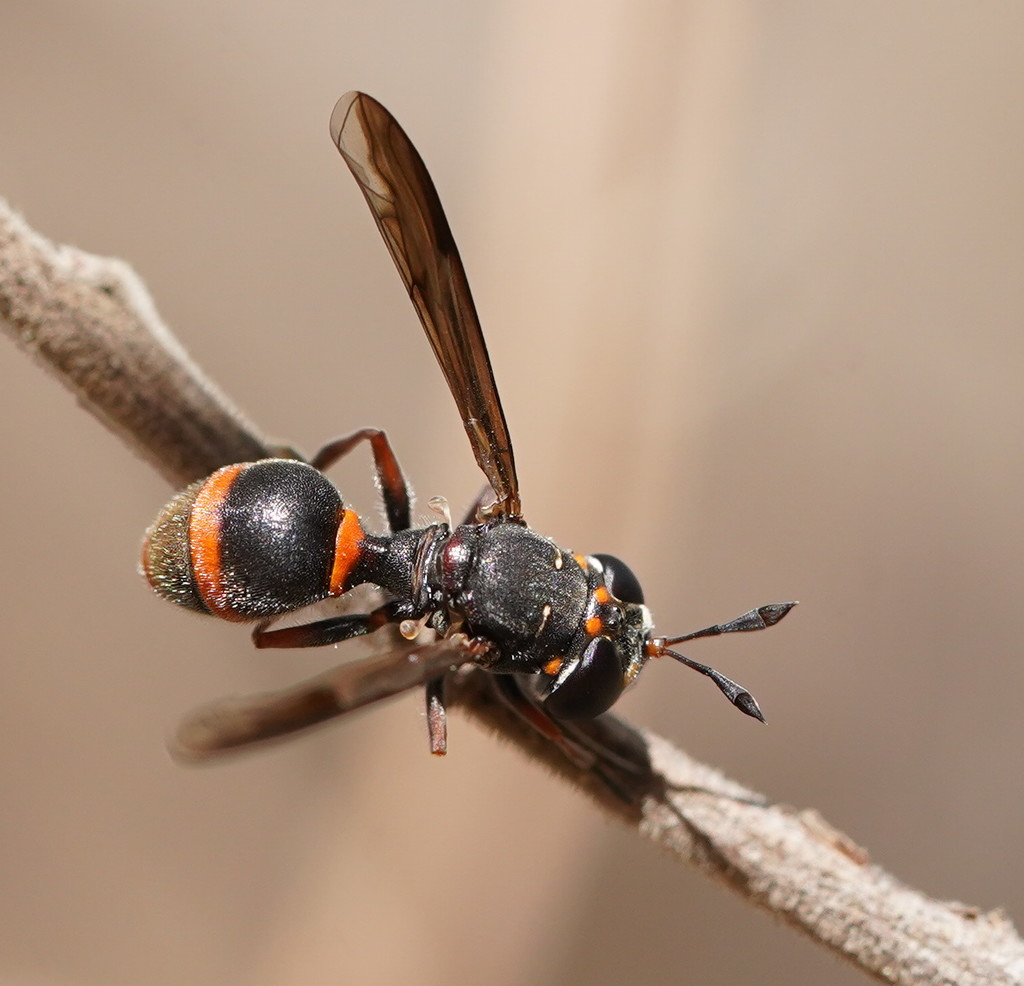In this high-quality, well-lit close-up image, a wasp rests on a diagonally positioned tree branch that stretches from the top left to the bottom right of the frame. The background is completely blurred, showcasing a light brown, furry texture that keeps the viewer's focus on the wasp. The wasp itself, positioned in the middle of the branch, is predominantly black, with its head facing the right side and its tail pointing to the left. It has two noticeable yellow-orange stripes across its bean-shaped tail, which transitions to a brown color at the end. The wasp's eyes are large and black, complemented by two short, blackish-brown antennae. Its pair of elongated brown wings, adorned with some black stripes, are visible and extend outward. While its front legs are not visible, its darker back legs are. There are orange circular dots near its black head, and some white fur is discernible on its back abdomen, adding to its detailed appearance.